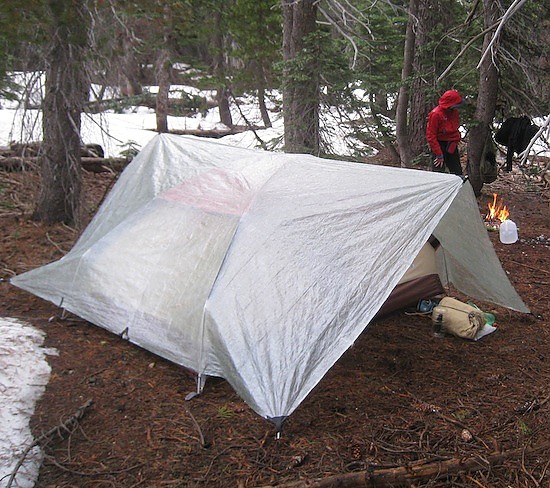In this detailed photograph taken in a wooded area, the ground is a rich blend of brown dirt speckled with fallen pine needles and discarded limbs. The left and right edges of the scene exhibit patches of snow, hinting at the cold temperature. Dominating the center, a small white tent, roughly four feet high, stands anchored on the dirt ground surrounded by brush. The tent, set up at an angle, features an opening on the right side, allowing a glimpse inside where some camping gear, possibly a sleeping bag and a cot, is visible. 

Beneath a larger tarp fashioned like an additional tent, this smaller tent provides a layered shelter experience. To the right, a figure in a heavy red coat with a hood and dark pants tends to a small fire. A clear, half-full, two-gallon plastic jug sits beside the fire, glinting in the flickering light. The backdrop is densely populated with trees, their trunks and branches framing the snowy ground that stretches further into the woods. The extensive detailing in the background includes more trees and snow-covered ground, creating a serene yet rugged camping scene. There appears to be an additional item, possibly a seat or chair, hanging off a tree behind the fire, adding to the lived-in feel of the campsite.